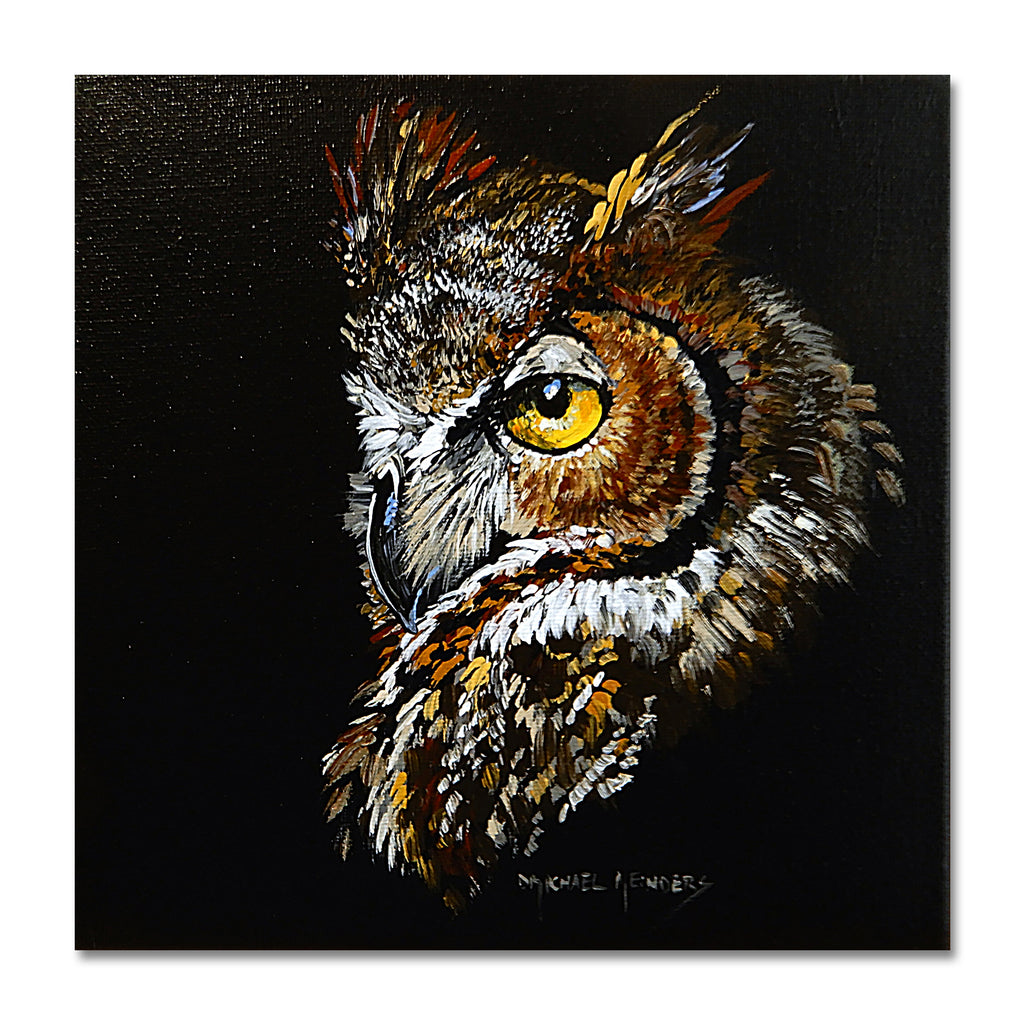This painting, likely an oil or acrylic piece by Michael Enders, portrays a stunning side view of an owl, possibly a great horned owl, against a deep black background. Dominated by rich shades of brown, golden yellow, white, and black, the owl's detailed feathers swirl impressively around its face, extending past its eye and in front of its dark, slightly blue-tipped beak. The captivating golden eye, with a distinct black pupil and white eyelid, commands attention as it gazes forward. The owl's head is slightly turned to the left, revealing part of its left shoulder and upright ear tufts while adding dimension to the composition. The upper left corner of the painting features white splotches, adding a textured, almost shiny contrast to the black backdrop. The artist's signature, "Michael Enders," is discernible at the center bottom of the piece.